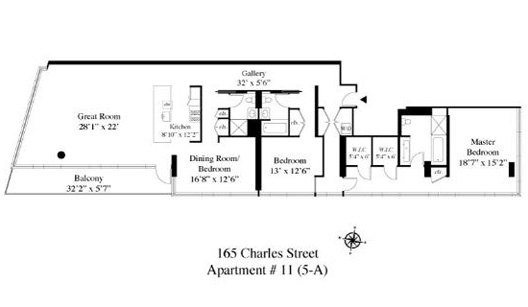**Detailed Caption:**

This image is a diminutive and low-resolution black and white floor plan schematic of an apartment. The simplicity of the diagram is characterized by clean line work. Below the floor plan, black text reads "165 Charles Street," followed by "Apartment Number 11" with "(5-A)" in parentheses on the subsequent line. To the right of this text, a faint compass logo can be discerned.

The floor plan outlines what appears to be a luxurious apartment. On the left side, there is an expansive "Great Room" measuring 28 feet 1 inch by 22 feet. Adjacent to the bottom-left corner of this room, a narrow "Balcony" stretches 32 feet 2 inches by 5 feet 7 inches. To the right of the Great Room, without any separating wall, is a "Kitchen" with detailed countertops and appliances, marked at 8 feet 10 inches by 12 feet 3 inches.

Above the kitchen, labeled "Gallery," is an area measuring 32 feet by 5 feet 6 inches. A thick line indicates a wall separating two bathrooms that share a common wall—each featuring a sink, counter, toilet, bathtub, and shower as seen from a top-down view. Below the left bathroom, a "Dining Room/Bedroom," measuring 16 feet 8 inches by 12 feet 6 inches, is identified. A thick line separates this space from an adjacent room labeled "Bedroom," which is significantly sized at 13 feet by 12 feet 6 inches.

To the right of the Great Room, a zigzagged hallway leads to two small square rooms labeled as "WIC," each approximately 5 feet 4 inches by 6 feet (the exact measurement is difficult to discern). Adjacent to these rooms, another small, unlabeled room resembling a bathroom is evident. This configuration is part of a long hallway.

At the far right edge of the floor plan, the "Master Bedroom" takes up a prominent square space, centrally marked with its name in black text. It is notably large, measuring 18 feet 7 inches by 15 feet 2 inches.

Overall, the floor plan illustrates a spacious and elegant apartment, with open spaces delineated by divider walls rather than solid room partitions, providing a sense of continuity and flow throughout the living areas.